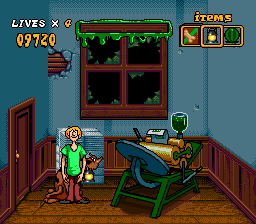Depicting a whimsical and slightly disheveled scene, the image is rich with eclectic details. On the left side, a weathered wooden door stands against a backdrop of vivid blue walls. Adjacent to the door, the lower portion showcases a stretch of brown wood. The upper background features a network of cracks, hinting at wear and age. To the center-left, brown branches sprawl out, adding a touch of natural chaos.

In the foreground, a peculiar window displays an unsettling patch of green goop, as if something untoward has happened. Near the middle of the scene, a green, shaggy chair draws one's eye, contrasting sharply with the comical figure of Shaggy, easily identified by his brown pants and distinctive orange hair, sitting or standing near it. Behind him, the loyal Scooby-Doo can be seen, adding an element of animated charm to the setting.

To the right, another green chair, this one equipped with yellow rollers, suggests a sense of functionality amid the clutter. Nearby, a jug filled with green liquid stands out alongside scattered papers and an enigmatic, large round object. Completing the curious tableau is a strange device, whose purpose is left to the viewer's imagination. This scene captures a playful yet mysterious atmosphere, teetering between the familiar and the bizarre.